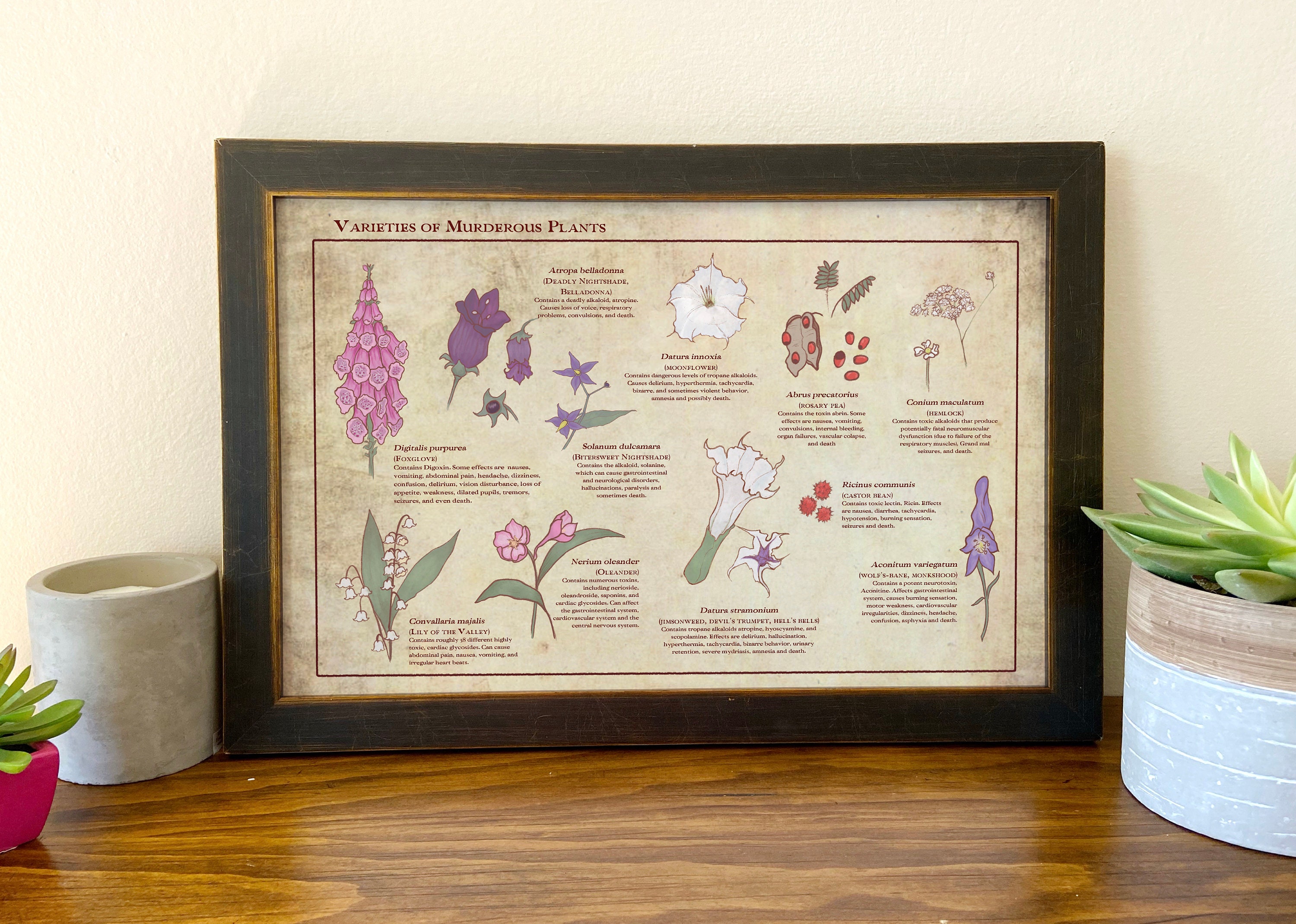The indoor image features a medium brown table adorned with darker brown striations creating a distinct pattern. On this table, there are two small plants. One, positioned on the right, is a succulent with yellowish-green, cactus-like petals held in a circular ceramic pot that is white at the bottom and brown at the top. The second plant has green stems with pink-tinged flowers held in a pink pot. Beside these plants sits a cylindrical gray candle with a visible white inner section.

Dominating the scene is a large, rectangular frame made from dark, natural-toned wood with an interior trimmed in a thin strip of gold. The frame displays a print titled "Varieties of Murderous Plants," resembling an instructional page perhaps from a book. The print features two rows of illustrations, each containing five images of various plants in shades of pink, purple, white, and red, complete with their names and brief descriptions.